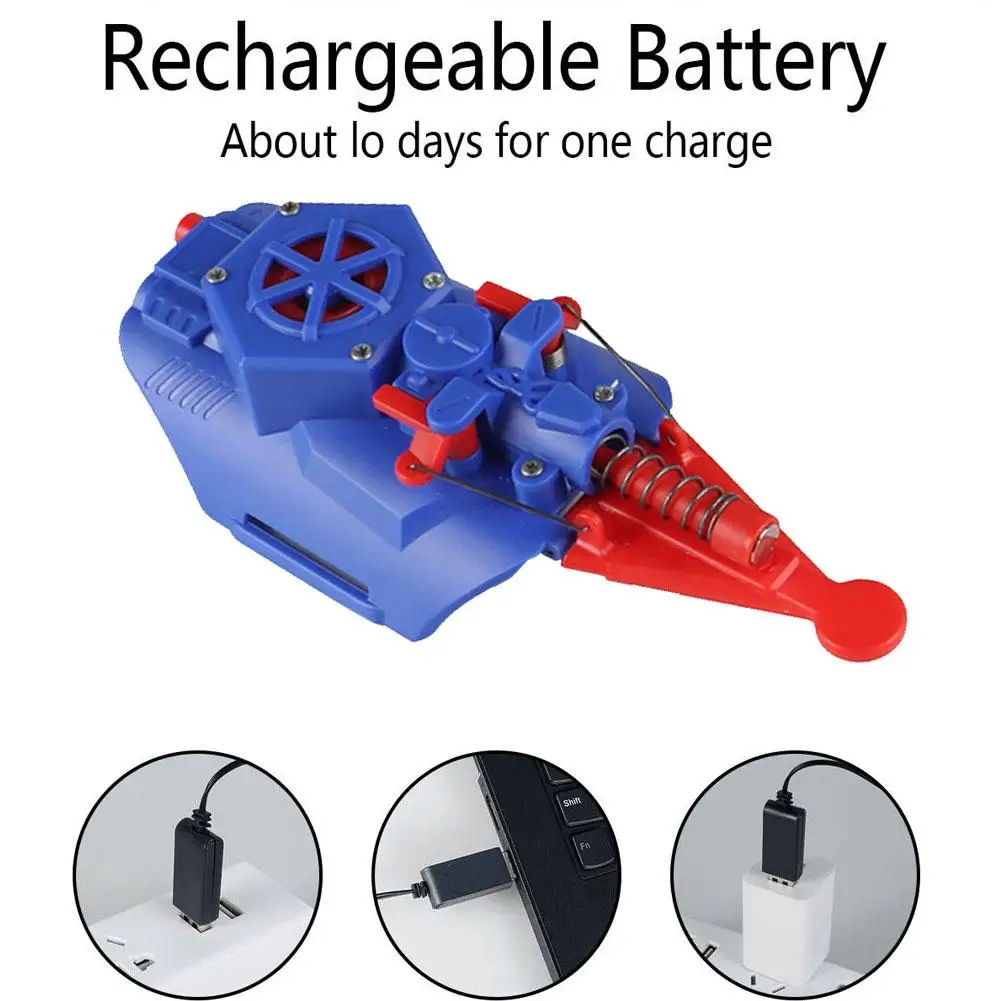The image features a white background with the text "Rechargeable Battery" at the top, indicating a charge lasting about "10 days" despite the text ambiguously showing "LO days." Dominating the center is a unique, compact plastic device resembling a miniaturized model of an engine or some mechanical component. This device is constructed with blue and red plastic parts, connected by screws and rivets, and includes a silver spring encased in a blue tube. The top portion of the device has a blue grille with a red inner area and a six-sided chamber, suggesting a vent or fan area. The lower half features a red triangular part with a round red tip. The bottom of the image depicts three circular icons illustrating a USB connection: one shows a USB plug being inserted into a socket, another into a laptop, and the third into a wall charger with a USB cable attached. The connection between the device and the USB icons is not immediately clear, but it's implied that the device can be charged using these USB methods.